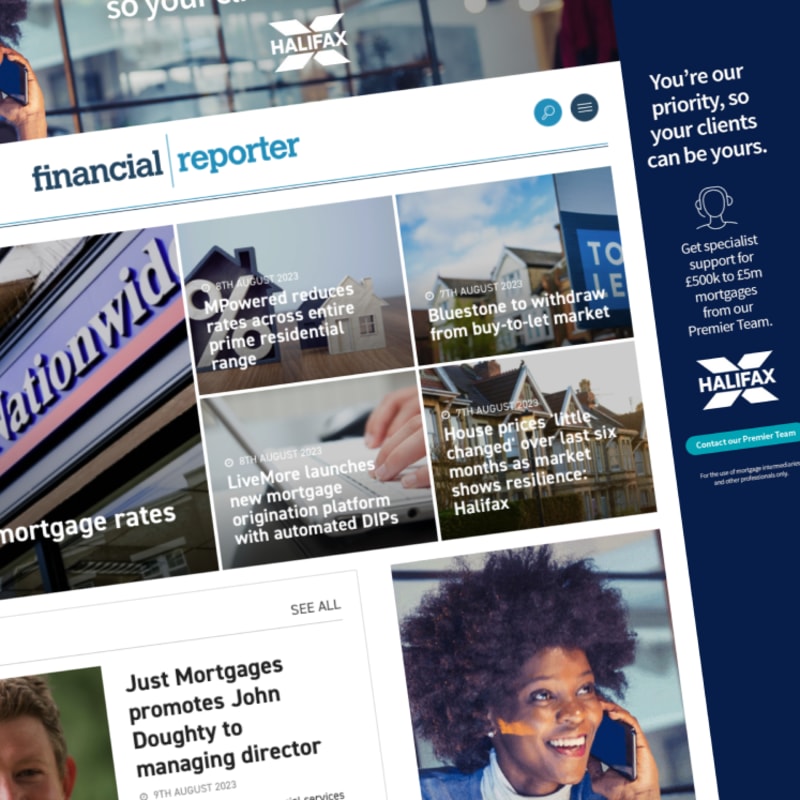This image captures a section of a website, slightly rotated to the left. At the top left, there is a photograph of a corporate office setting, where only a person's hand holding a mobile phone is visible on the left. Central to the image is a prominent white 'X' logo with the word "Halifax" in white capital letters running through the middle. Beneath this logo is a white background.

In the top left corner, the word "financial" is written in dark blue, followed by a thin blue vertical line. To the right of this line, the word "reporter" appears in light blue. There is negative space to the right, which is followed by a teal blue circle containing a white magnifying glass icon. Adjacent to this is a dark blue circle with three horizontal white lines stacked vertically, functioning as a menu icon.

Below the header, a decorative underline is composed of a light blue squiggly line on top and a gray squiggly line beneath it. The content area consists of multiple panes featuring images and text. The prominent image on the left showcases a blue sign with white text stating "nationwide," and at the bottom, partially visible words "mortgage rates." 

To the right of this main image is a two-by-two grid displaying four smaller pictures. Three of these images feature houses, while the bottom left image displays a white laptop. Accompanying these images are the following text snippets, from left to right and top to bottom:
1. "Empowered reduces rates across the entire prime residential range."
2. "Bluestone to withdraw from buy to let market."
3. "LiveMore launches new mortgage origination platform with automated DIPs."
4. "House prices little changed over the last six months as market shows resilience Halifax."

Beneath these images, there is additional content on a white background, which includes text and images. On the far right, a blue sidebar contains white text, though specific details of the sidebar content are not clearly described.